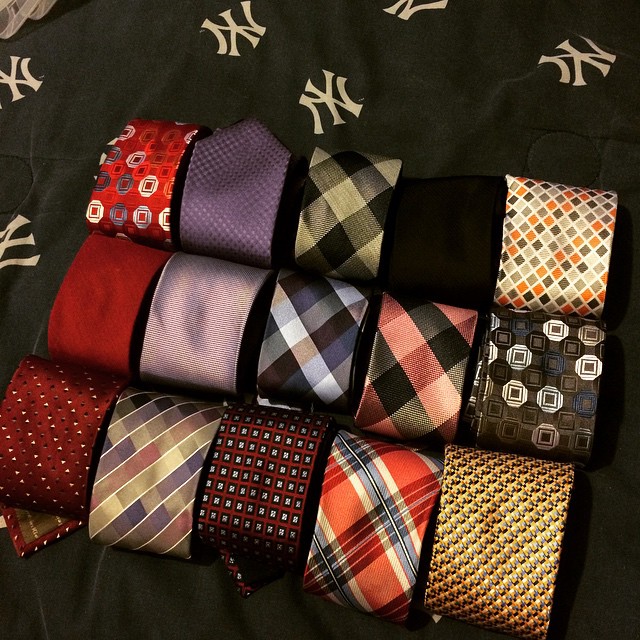This color photograph taken from above showcases a neatly arranged display of 15 rolled men's neckties on a dark background adorned with the iconic New York Yankees logo in white. The ties are organized into three rows, each containing five ties, and they are meticulously rolled, exposing around four inches of each tie’s length. Their shimmering fabrics, likely silk, satin, or nylon, exhibit a range of vibrant and muted colors along with various intricate patterns.

The ties positioned in the top row include:
1. A red tie with white and gray geometric designs.
2. A blue tie featuring a lighter blue pattern.
3. A black and white plaid tie.
4. A solid black tie which subtly blends into the black background.
5. A tie with a small checkerboard pattern in red, black, gray, and white.

In the middle row, from left to right, the ties are:
1. A solid brick red tie.
2. A blue tie with subtle wavy white lines.
3. A blue, black, and light blue plaid tie.
4. A red and black plaid tie.
5. A gray tie with black, blue, and white geometric patterns reminiscent of the first tie but with different colors.

The bottom row features:
1. A maroon tie with diagonal stripes formed by small polka dots.
2. A tie with diagonal lines in muted mauve, purple, and tan color blocks.
3. A red tie with small white squares outlined in black or dark blue.
4. A red, white, and blue plaid tie.
5. A gold tie featuring a herringbone pattern or texture.

These ties rest on a New York Yankees blanket, distinguished by the repeated N and Y logo, adding a sporty yet elegant backdrop to this sophisticated array.